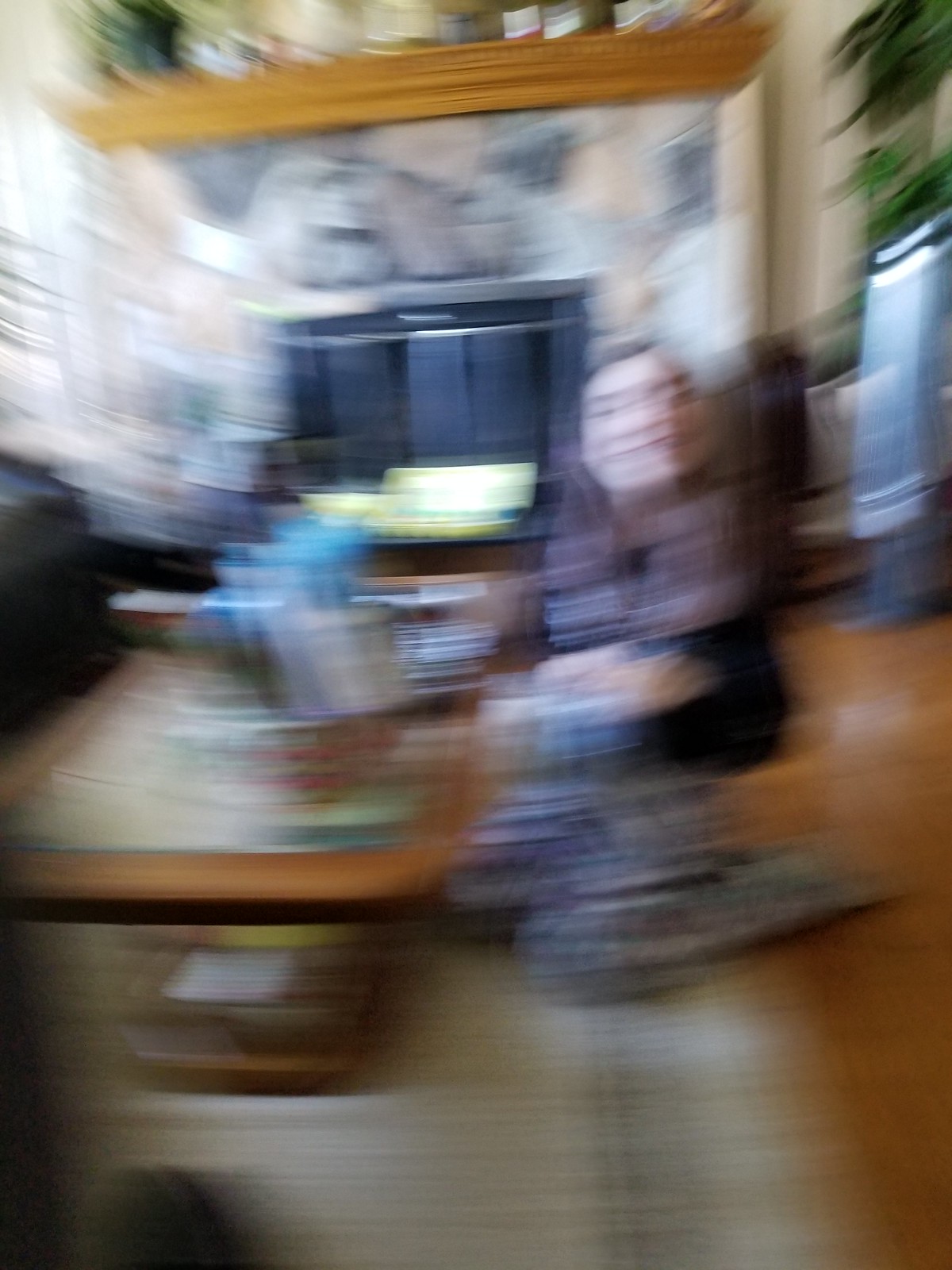This is an extremely blurry photograph of what appears to be a young girl kneeling on a rug in front of a rectangular wooden coffee table with a possible glass center insert. The setting includes hardwood flooring around the rug and a fireplace with a stone facade and a wooden mantel in the background. The tabletop is cluttered with various items, showing hints of red, blue, and white colors, although the specifics are indiscernible due to the poor image quality. The girl, who seems to have short hair, is looking towards the camera, possibly smiling. The scene also includes a black fireplace with a silver outline and assorted objects on the mantelpiece that are not clearly identifiable.